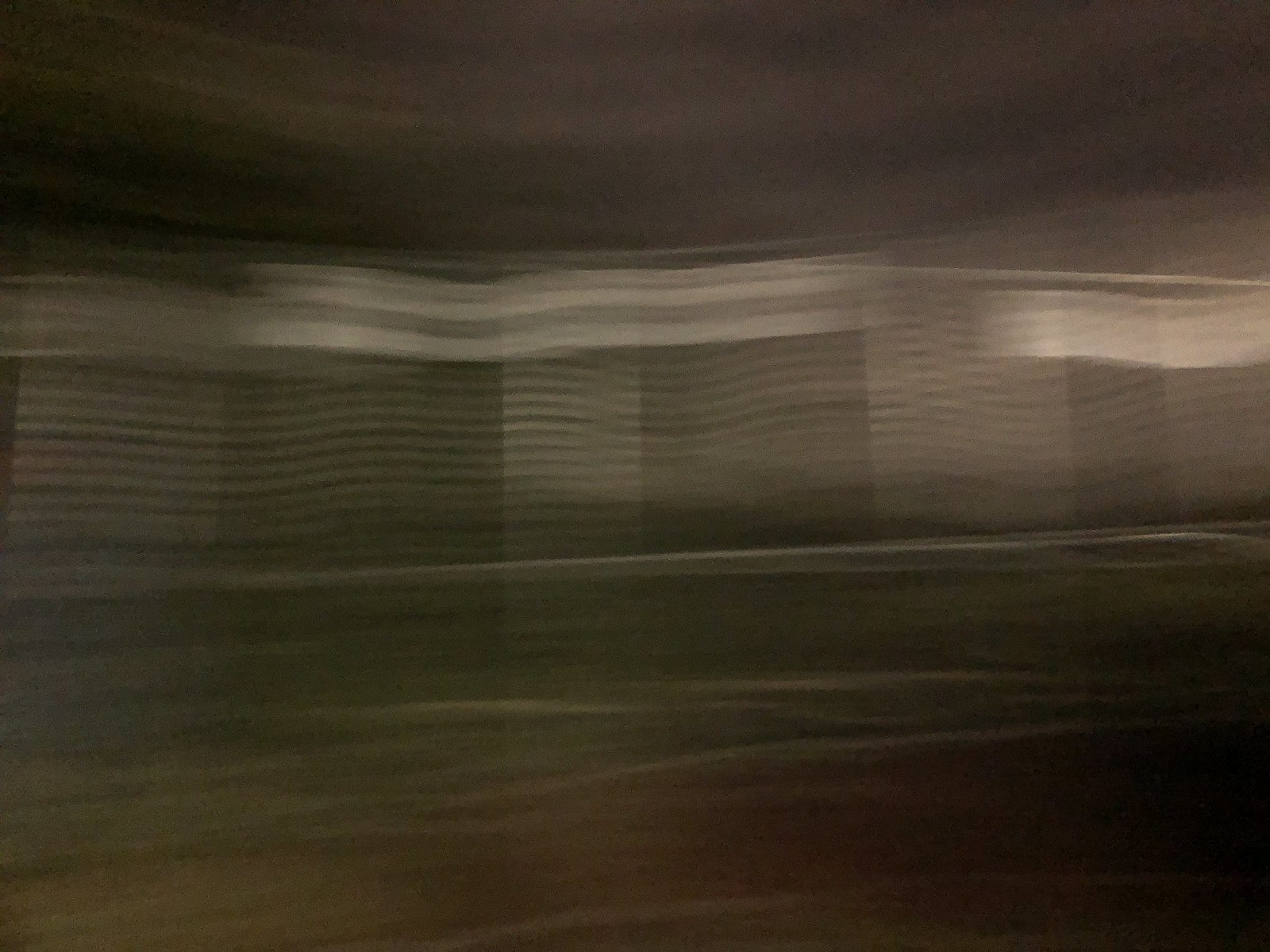An abstract image characterized by its non-representational elements features a dominant palette of varying shades of gray interspersed with hints of color. The upper section is primarily occupied by a deep blue-gray expanse, setting a somber tone. Directly beneath this area, a band of alternating light and dark stripes stretches horizontally from edge to edge, creating a stark contrast with the darker hues above. These stripes, composed of white and gray lines, add a rhythmic pattern to the composition. Below this central band, a wave-like form of soft gray curves gently across the width of the image, creating a sense of depth and movement. This lower portion is interspersed with a few delicate white lines, adding subtle highlights and further enhancing the image's dynamic nature.